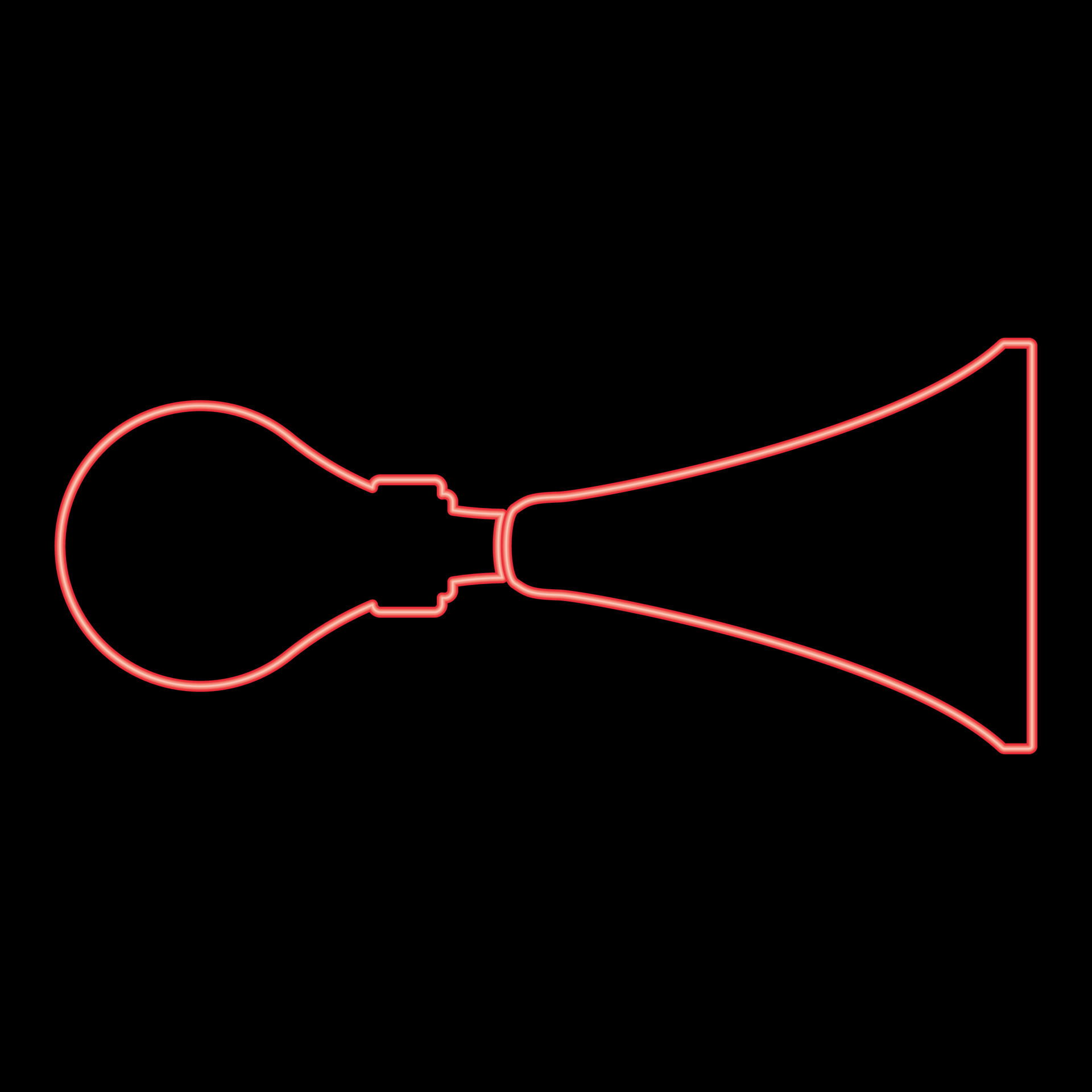The image depicts a large black-filled square featuring a distinct neon-lit outline in a glowing pinkish-orange color. The outline resembles a combined shape: on the left, there's a figure similar to a classic bicycle horn with a bulbous end, and on the right, it transitions into a cone shape, akin to a megaphone. This continuous neon outline gives the impression of a light or neon sign, with a thin yellow line running through its center, enhancing the glowing effect. The background is completely opaque, providing a stark contrast to the vibrant, holographic lines that form the unique object.